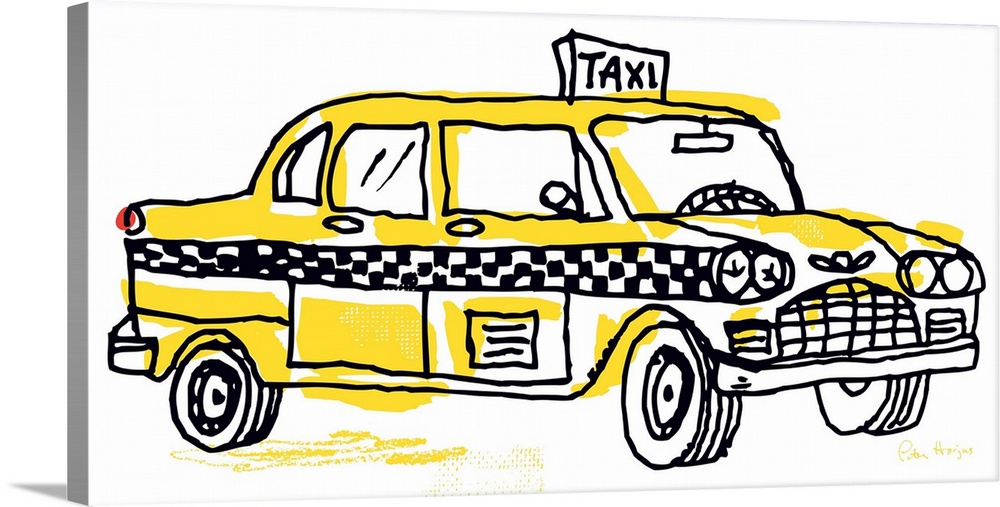This image features a highly stylized, cartoonish illustration of a New York City taxi cab on a white canvas. The artwork resembles an ink drawing with playful, imperfect coloring that doesn't stay within the lines. The taxi is predominantly highlighted in yellow with a distinctive checkered stripe running down its side, and there are additional splashes of color, including a touch of red on the taillight. Detailed elements like the steering wheel, headlights, three visible tires, brake lights, rearview mirror, and side mirror are all present. A traditional "TAXI" sign sits atop the cab. The illustration is either done on a canvas or a digital representation mimicking a canvas, with a slight shadow cast on the left side. The artist's name, possibly Peter Hargis, is signed at the bottom right in yellow, though it is somewhat difficult to decipher.